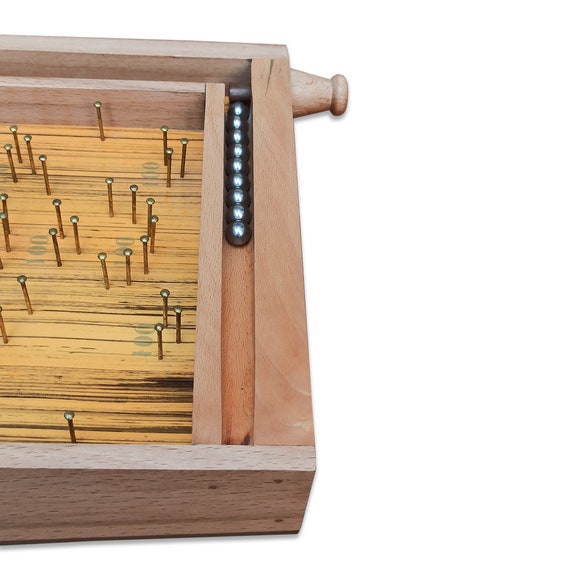The image showcases a primitive version of a pinball machine against a plain white background, possibly digitally altered with a fake drop shadow to enhance its presentation. The pinball machine, cropped tightly in a portrait orientation, reveals only its bottom portion where one might pull the lever to launch the ball. The structure is wooden, featuring a simple design primarily made from unstained wood, potentially pine, with a smooth, flat surface. The backboard, however, contrasts with a stained finish, emitting a yellow hue, suggesting a decorative touch.

The machine's interior is minimalist, populated with several metal pins standing erect on the lightly colored wood. Scoring markers, such as "100 points," are inscribed near specific slots or crevices where the ball can land, implying a scoring system. Nine silver balls are queued in a carved-out area within the box, ready to be deployed. A wooden handle, described as resembling a short antenna, protrudes, likely used to release the balls. The set-up suggests that the ball, once launched, navigates through the arrangement of pegs or pins, resembling a rudimentary yet functional and engaging game mechanism.